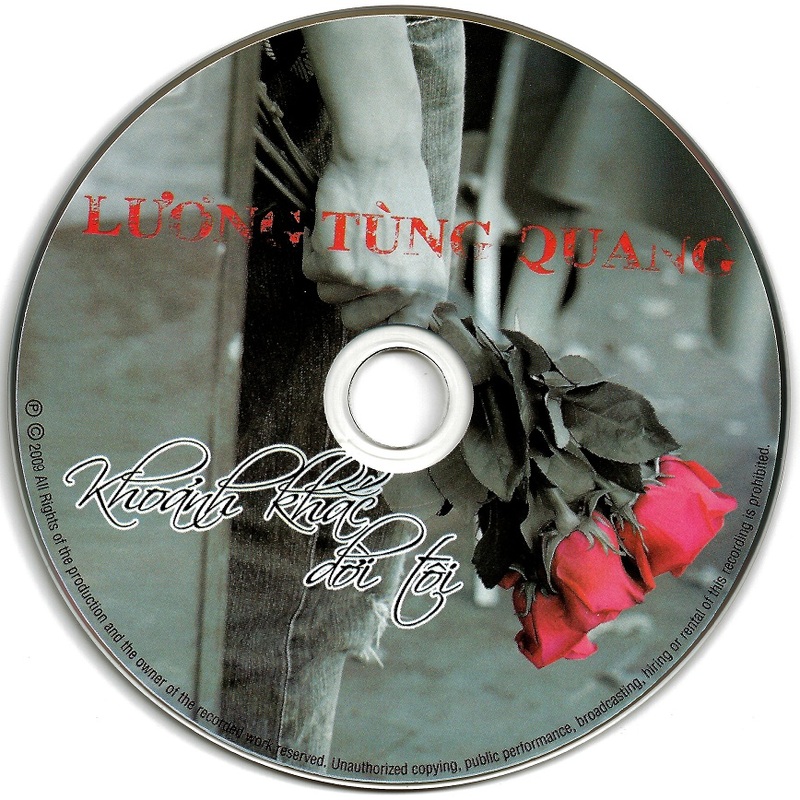This photograph features a round CD adorned with a striking black-and-white image of a boy in jeans, holding a bouquet of vibrant red roses by his leg. The boy is leaning against the exterior wall of a building, creating an evocative scene. The composition is largely in black and white, making the red rose petals stand out vividly. Red text, presumably the artist's name in Vietnamese, "Luon Tung Kwong," is prominently displayed about a third of the way down the CD. Below this, black text, also in Vietnamese, likely indicates the album title, "Kwong Kak Doi Toi." The bottom rim of the CD includes a copyright notice stating, "© 2009 all rights of the production and the owner of the recorded work reserved. Unauthorized copying, public performance, broadcasting, hiring or rental of this recording is prohibited."